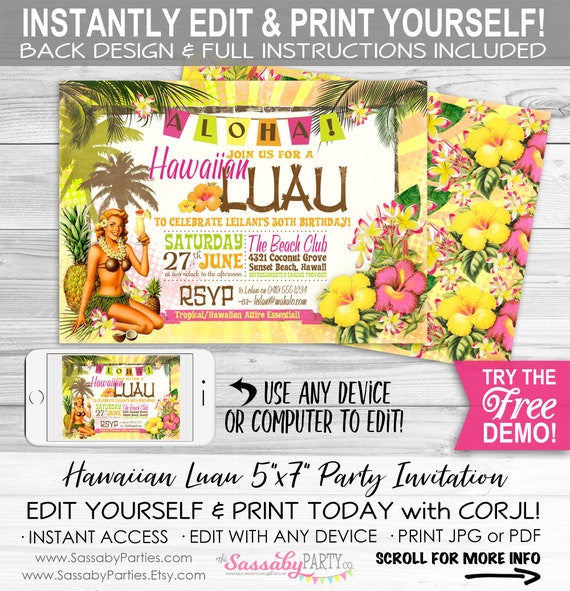This image features a detailed mock-up showcasing an editable and printable invitation for a Hawaiian-themed luau. The top section displays a gray rectangular banner with the text "Instantly edit and print yourself. Back design and full instructions included," written in white. Below this banner is a textured gray wooden surface that serves as the background for the vibrant invitation.

The invitation itself is eye-catching and colorful, designed to evoke the tropical spirit of Hawaii. It prominently features an assortment of yellow and pink flowers, green leaves, and pink and white flowers to create a lively, floral border. The word "Aloha" is highlighted at the top in multicolored banners of pink, green, and yellow, setting a festive tone.

Text on the invitation reads, "Join us for a Hawaiian luau to celebrate Leilani's 30th birthday," with the event scheduled for Saturday, 27th of June. An RSVP section instructs guests to respond, and the venue is listed as "The Beach Club," vividly noted in pink.

A smiling lady dressed in traditional Hawaiian attire, including a coconut bra and a lei around her neck, is prominently featured. She is holding a drink and stands in front of a pineapple, adding to the cheerful and festive Hawaiian theme of the invitation.